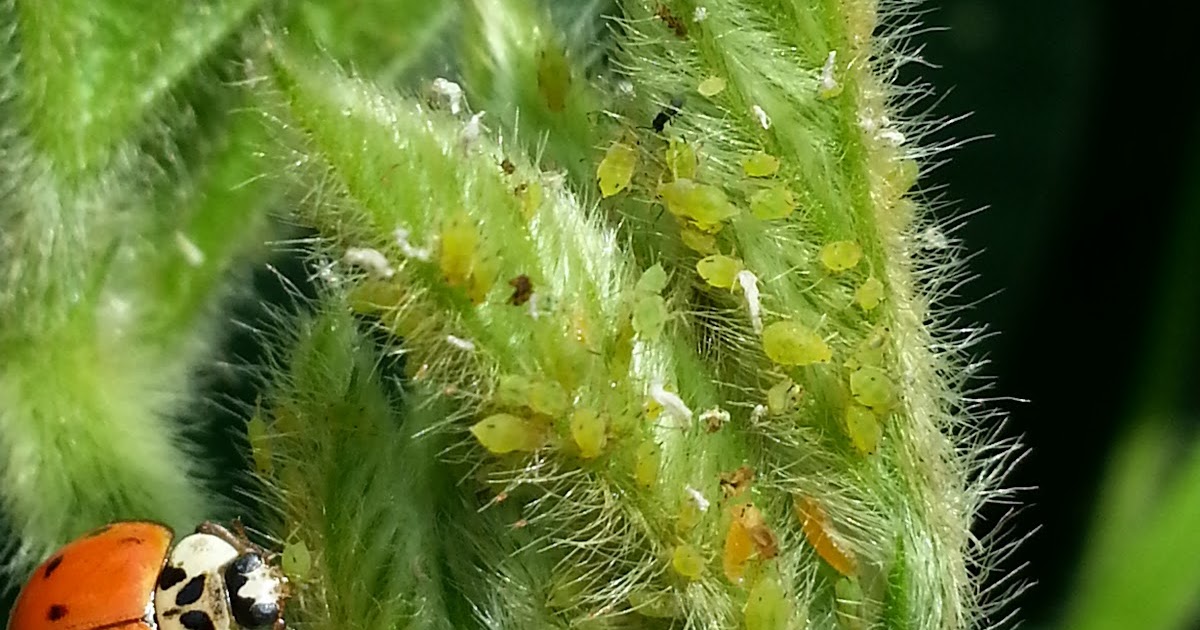This image is a detailed close-up photograph of green, feather-like plants, possibly cacti, taken outdoors. In the center-right of the image, the plants are in sharp focus, showcasing white, hair-like follicles that contrast with the green central stems. These plants extend off the image at both the bottom and the right edges. The leftmost plant curves upwards and to the left, staying within the frame and displaying fewer green pods compared to the one on the right. In the background, more of these green plants are visible but blurred, creating a depth effect. The right side of the image fades into a mix of dark and light green colors. In the bottom left-hand corner, there's a prominent ladybug, partially cropped by the edge of the frame. The ladybug has an orange-red back with black spots, and a distinctive white head marked with black. It seems to be climbing on the plant and appears to be feeding on tiny green bugs, likely aphids, which are abundantly scattered over the plant’s surface. The far right background is primarily dark, with occasional green hues that hint at more foliage.